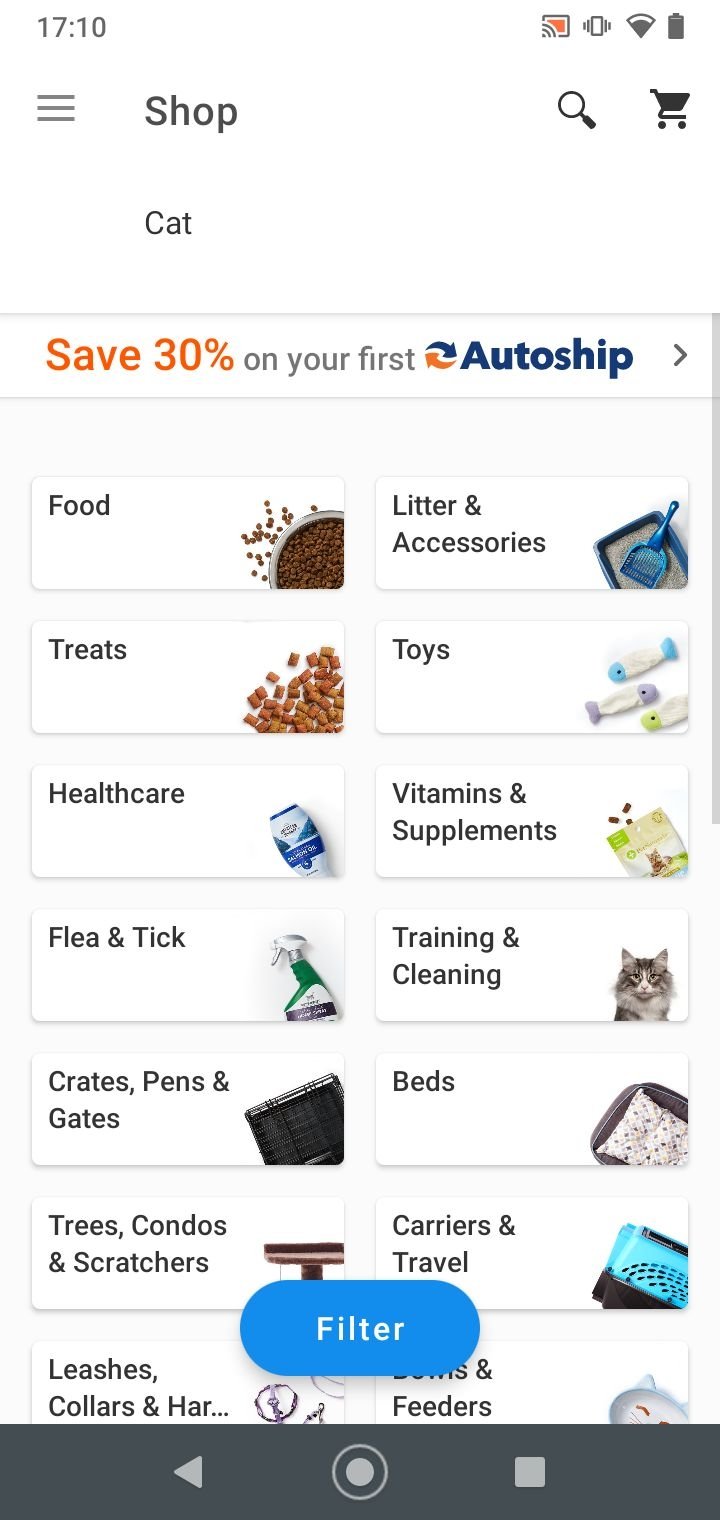The screenshot captures a shopping application displayed on a smartphone. The orientation of the screenshot is vertical, with the sides significantly longer than the top and bottom edges. The very top portion of the image is white, seamlessly blending the app's interface with the phone's UI elements. In the top left corner, the time is shown as 17:10. On the top right, a series of icons are present: a simulcast symbol, a vibration symbol, a connectivity symbol, and a battery icon.

Just beneath the UI, the application title "Shop" is prominently displayed in black text, accompanied by a black magnifying glass icon for search functionality and a black shopping cart icon for cart access. Below this title, the word "Cat" is displayed on a white background, suggesting the section or category within the app.

The app presents several categories for the user to choose from, organized neatly in two columns. Above these categories is a white banner with a promotional message stating, "Save 30% on your first auto-ship."

Each category is denoted with black text paired with a corresponding image. Starting from the top left and moving right, the first category is labeled "Food" and is illustrated with an image of a silver bowl filled with brown kibble. To its right, another category is marked "Litter & Accessories," though the associated image is partially cut off in the description provided.

Overall, the screenshot offers a clear view of the shopping app's user interface, with easy navigation options and promotional offers intended to attract and assist the user.